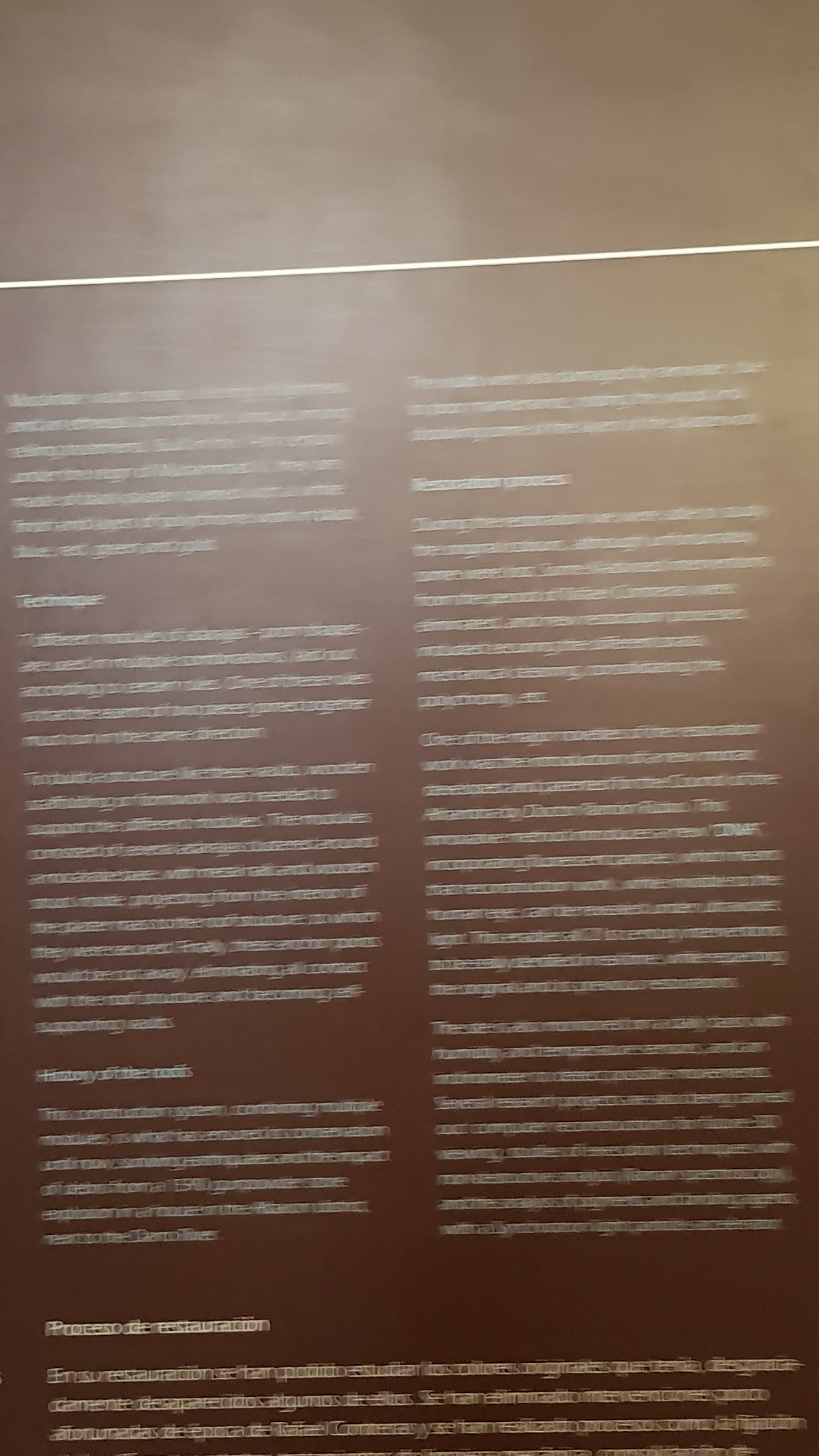The image features a vertically rectangular, glossy brown page, slightly mixed with light gray at the top left. Approximately an inch from the top, a thin white horizontal line stretches across the page. The primary content consists of small, blurry white text organized into two vertical columns, each containing four paragraphs. Below these, there's an additional paragraph spanning the entire width of the page. Although most of the text is unreadable due to the blur, the second paragraph appears to be titled "Telescope", and the following one is "History of the Roads." Overall, the page contains a total of eight paragraphs in columns and one wide paragraph at the bottom, all set against the consistent brown background.